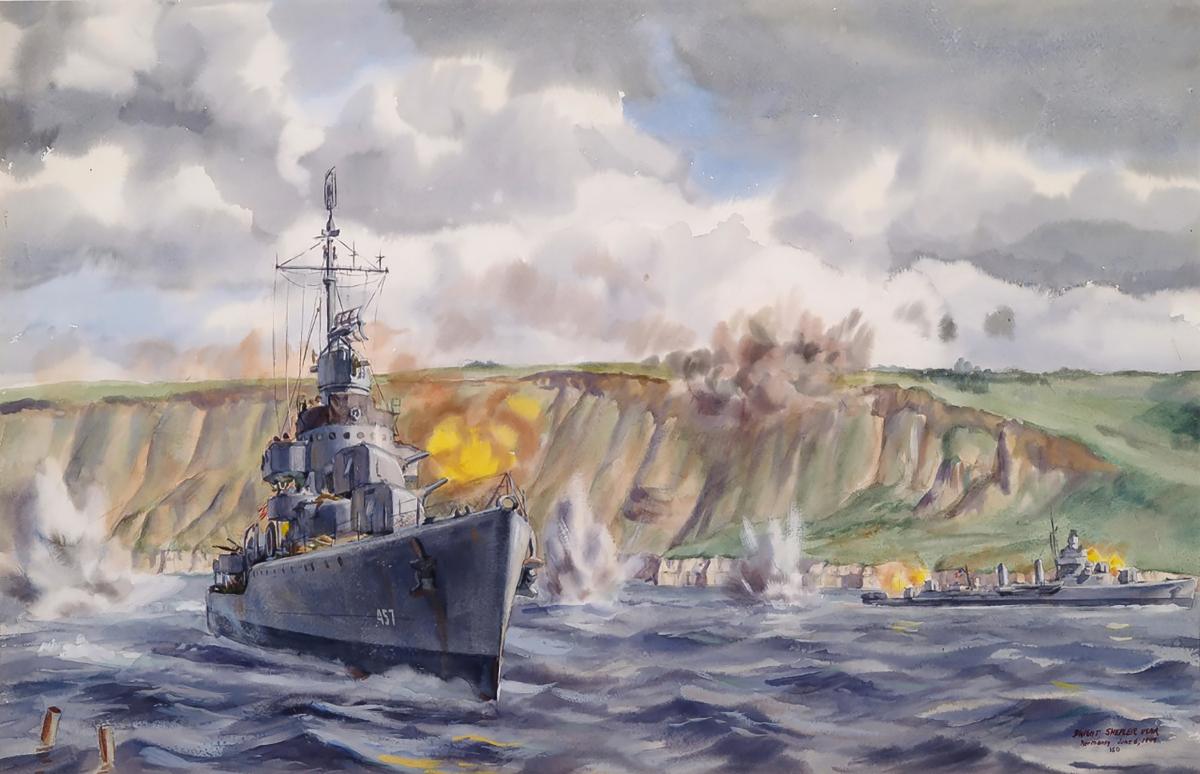The painting depicts a dramatic wartime scene, rendered in a watercolor-esque style, capturing the intensity of naval warfare. Dominating the foreground is a large, gray battleship, reminiscent of those from World War II, with an elongated body, a pointed prow, and a central tower bristling with gun turrets and antennae. It cuts through choppy blue waters, creating a sense of motion and urgency.

Around the battleship, the water is disturbed by numerous splashes from artillery shells, with bright yellow muzzle flashes illuminating the scene. To the left, flames rise ominously above the vessel, while another ship can be seen in the distance on the right, possibly beached and on fire, adding to the chaos.

The backdrop is a tan, green-covered hillside, featuring brown cliff-sides and grassy tops. The sky overhead is filled with dense, gray clouds, enhancing the painting's somber and turbulent atmosphere. Explosions and sprays of water suggest a fierce exchange of fire, with the destroyer shelling the shoreline and return shots hitting near the ship. Despite the violence, the loose and vivid watercolor technique imbues the scene with a poignant, almost surreal quality.